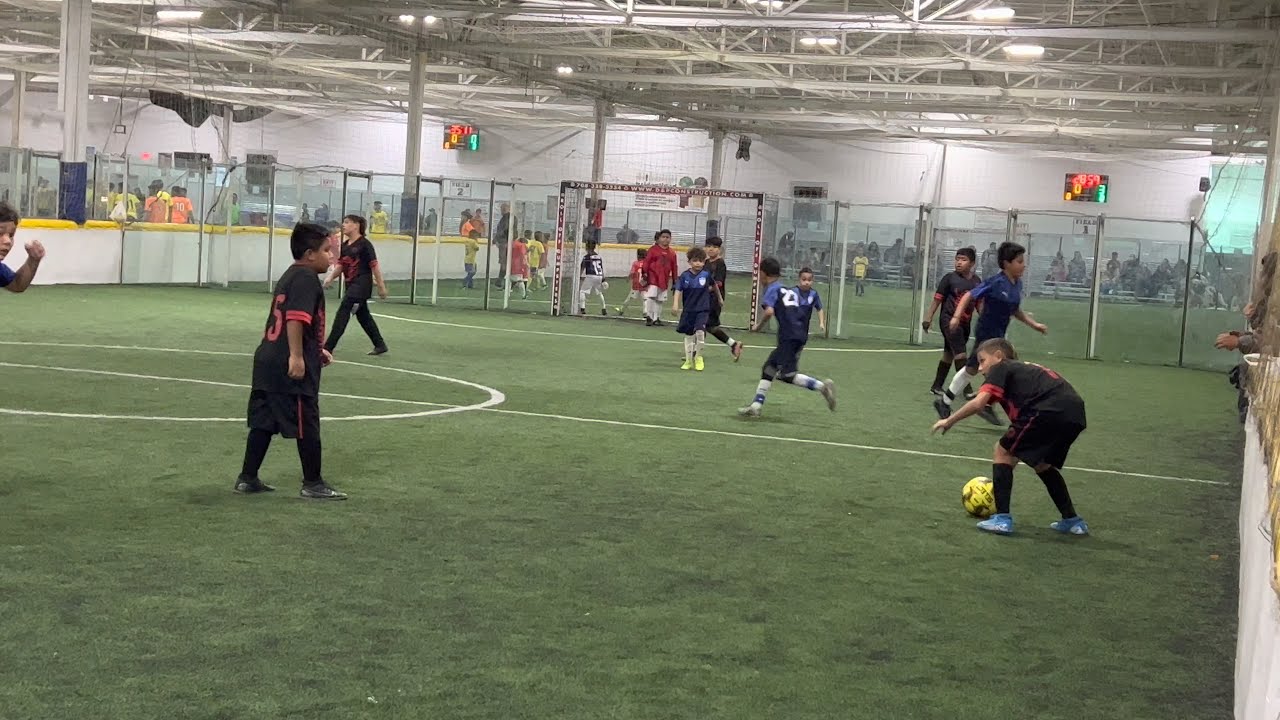This image depicts an indoor soccer arena filled with young children playing soccer. In the foreground, the focus is on a player in a black jersey with red numbers, hunched over, ready to kick a yellow soccer ball to his teammate. His team faces another wearing black jerseys with blue shoulders, one of whom sports the number 23 on his back. The game takes place on a green surface, likely artificial turf, considering the indoor setting. The arena's white walls are lined with a white fence topped with yellow. Overhead, industrial lights and steel rafters illuminate the scene. Scoreboards against the back walls display the time and scores, while several white columns support the roof. Behind the fences, people in orange shirts, possibly coaches, can be seen. The setting and dynamic energy conveyed suggest an engaging soccer match featuring determined, pre-teen players.